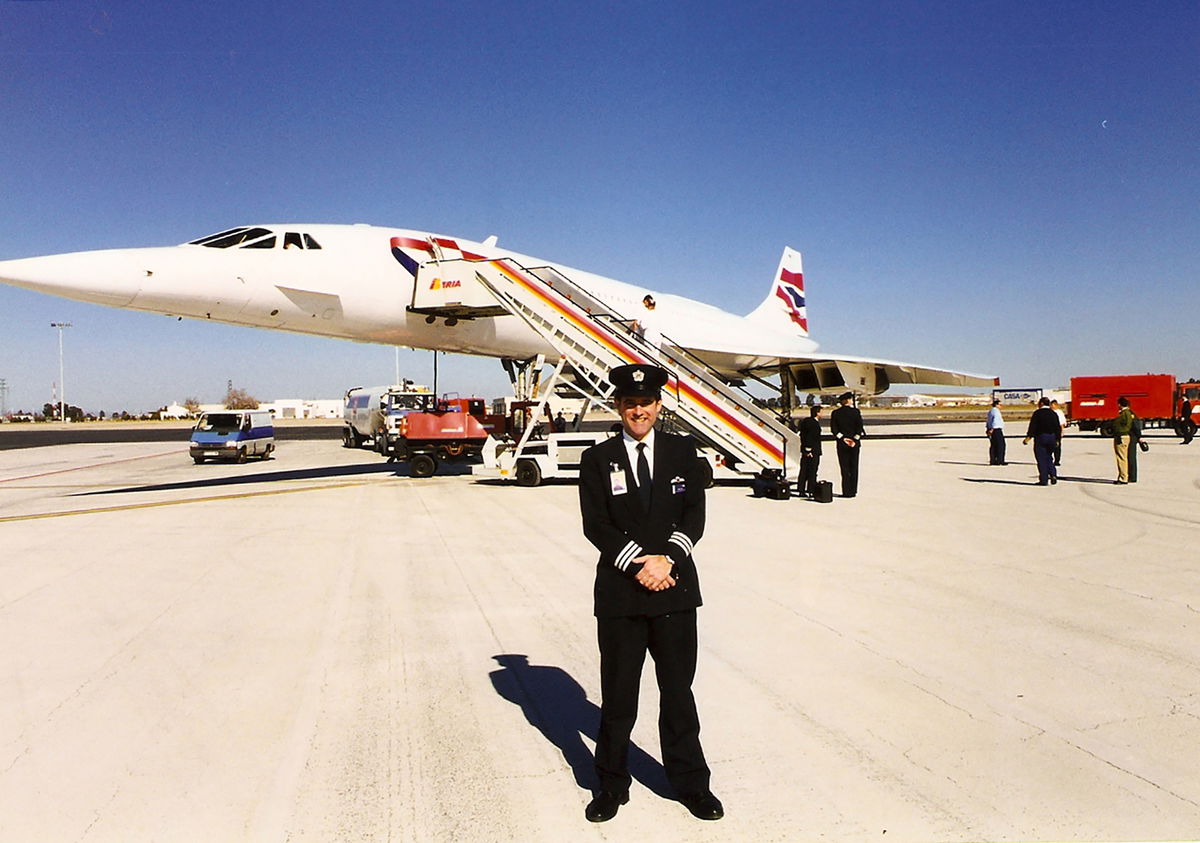In this bright midday photograph, we see a prominently featured Caucasian pilot in a polished black uniform with three white stripes on each cuff and a black hat adorned with a badge, standing front and center, smiling confidently with his arms crossed. Behind him, a high-tech, white jet with a highly pointed nose reminiscent of a fighter jet is positioned diagonally, approximately at an 8:30 angle. The jet features a red and yellow striped exit ramp extending from its mid-side front left. 

In the foreground, several airport and flight personnel are visible, conducting various activities around the jet. There are vehicles such as a blue and white bus parked under the aircraft, a red semi-truck in the distance, and what appears to be a white oil truck with blue text, though the text is indistinguishable. A smaller red construction vehicle can also be seen beneath the plane. A staircase descends from the jet, with a man dressed in white walking down. 

In the background, set against the blue sky, are additional flight personnel, including pilots with luggage, and a distant white building with lampposts visible against the clear horizon, contributing to the busy yet orderly atmosphere of the airport scene.